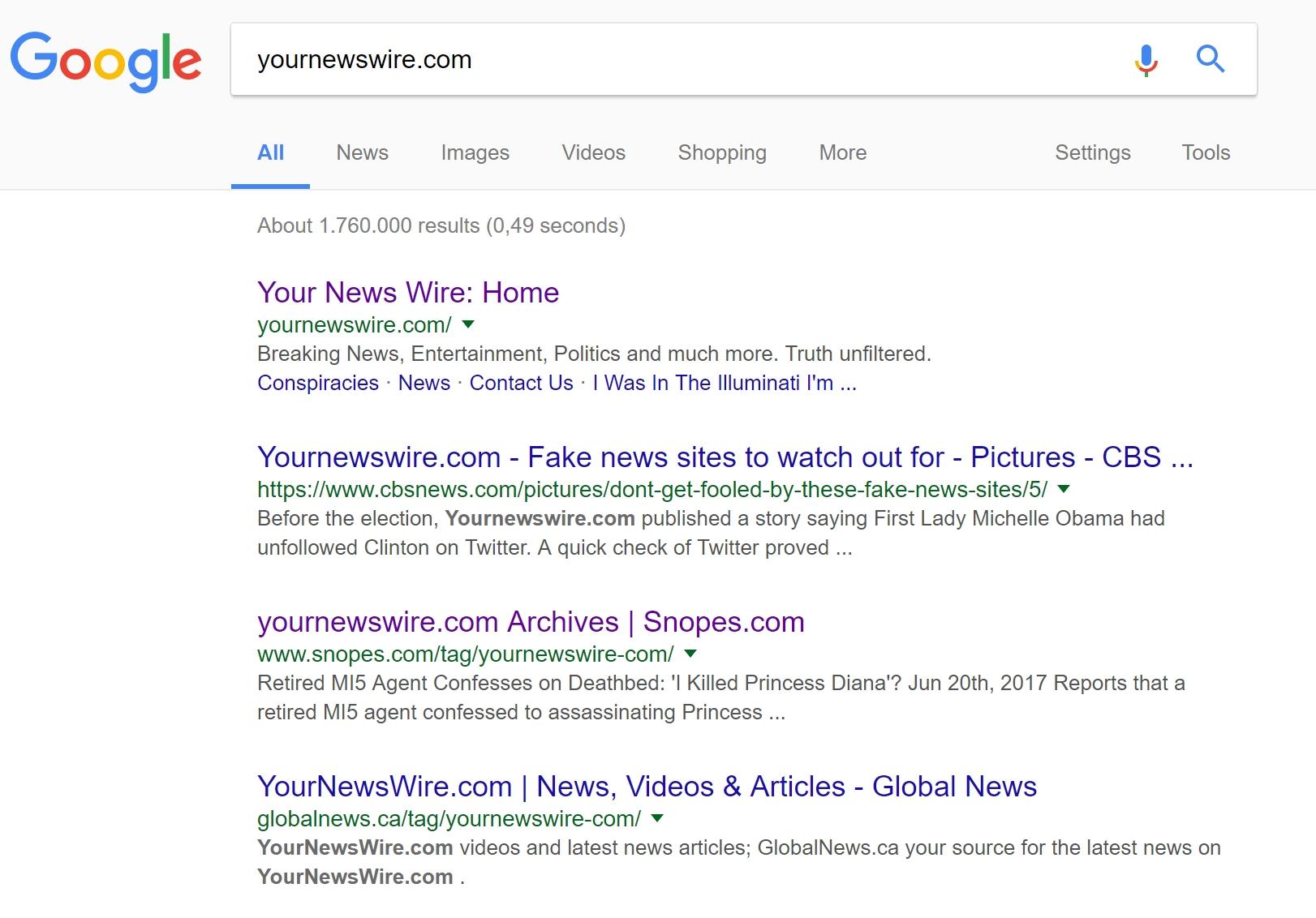**Search Results on "Googly" for YourNewsWire.com**

The image displays a search results page from "Googly," showcasing the search query "yournewswire.com" in the search bar. The "Googly" logo, featuring its signature blue, red, yellow, and green colors, is situated in the top-left corner of the page. 

Below the search bar, various search categories are listed: All, News, Images, Videos, Shopping, Malls, City, and Food. The search results indicate about 1,260,000 results obtained in 0.49 seconds.

**First Result:**
- **Title:** yournewswire.com (in purple, indicating a previously clicked link)
- **URL:** yournewswire.com (displayed in green)
- **Description:** "Breaking news, entertainment, politics, and much more; truth unfiltered."
- **Sub-categories:** - Conspiracies
                   - News conductors
                   - I wish I was in the Illuminati
                   - Knows where I am
                   - Blue card

**Second Result:**
- **Title:** yournewswire.com Fake News Sites Watch Out For (in blue)
- **URL:** cpsnews.com
- **Description:** "Before the election, yournewswire.com published a story claiming First Lady Michelle Obama had unfollowed Clinton on Twitter. A quick check on Twitter proved [incomplete]."

**Third Result:**
- **Title:** yournewswire.com Archives
- **URL:** snopes.com
- **Description:** "Retired MI5 agent confesses on deathbed: 'I killed Princess Diana.' June 2017 report stated a retired MI5 agent confessed to assassinating Princess Diana."

**Fourth Result:**
- **Title:** yournewswire.com News Videos and Articles
- **URL:** globalnews.ca
- **Description:** "Yournewswire.com, videos and latest news articles. Globalnews.ca, your source for the latest news on yournewswire.com."

The background of the webpage is predominantly white, adhering to a clean and straightforward aesthetic.